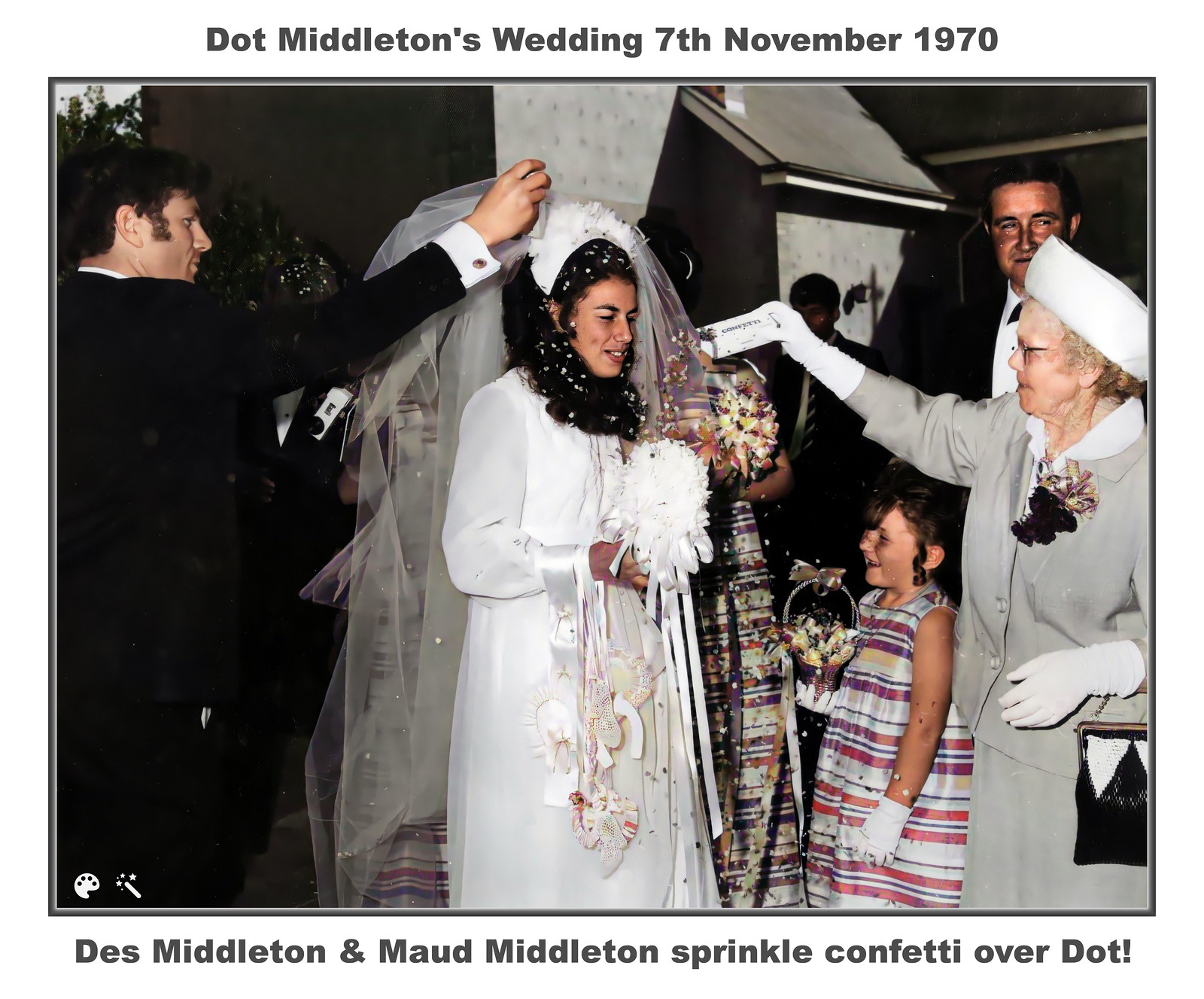Set against a white background, this photograph captures a joyous moment from Dot Middleton's wedding on November 7th, 1970, as indicated by the black text above the image. Below the photograph, a footnote reads, "Des Middleton and Maude Middleton sprinkle confetti over Dot." The bride, Dot, stands in the center, looking to the right from our perspective. She has long dark hair cascading under a white veil that flows down her back. Wearing a long-sleeved white wedding dress and holding a white bouquet, Dot is the focal point of the scene.

To Dot's left, Des Middleton, a young man with black hair, wearing a black suit and a white shirt—his cufflinks visible—is in the act of raising his right hand to sprinkle confetti on the bride. On Dot's right, Maude Middleton, an elderly woman adorned in a gray dress, white hat, black brooch, white gloves, and holding a black purse, is also showering the bride with confetti.

Additionally, a little flower girl stands between the bride and Maude. The child is dressed in a white outfit with purple and pink stripes, and she holds a small basket of flowers and wears white gloves, joyfully smiling at the confetti shower. The scene appears to be outdoors, with the exterior of a gray-walled building and some greenery visible to the left, suggesting it might be near a church. Behind the main subjects, more people can be seen, including two bridesmaids in multicolored dresses and men in dark suits, adding layers of depth to this celebratory wedding moment.